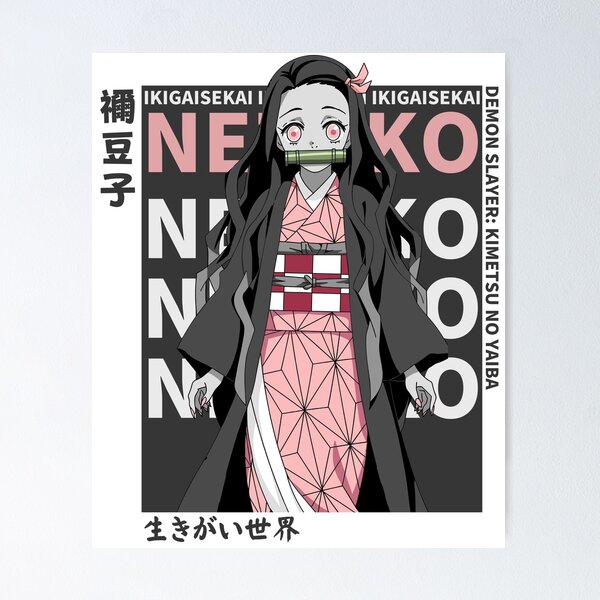The image is a detailed poster featuring Nezuko from the anime "Demon Slayer: Kimetsu no Yaiba." The poster has a light gray background with a gray square shape, and within it, a smaller white rectangle positioned vertically. Surrounding the main image, there are Japanese characters and the text “Demon Slayer: Kimetsu no Yaiba.”

Nezuko, depicted in the animation style typical of anime, is the central figure. She has long black hair adorned with a pink ribbon. Her eyes are pink with distinct irises, and she gazes directly at the viewer with a somewhat vacant expression. Covering her mouth is a cylinder-shaped, metallic green object that resembles a container for a small scroll or a piece of bamboo.

She is dressed in a pink kimono decorated with geometric designs, and over it, she wears a nearly black, dark gray robe. The kimono is fastened by a thick rectangular belt with a white and red checkerboard pattern just below her chest. Her hands, visible within the frame, display sharp, pink-colored nails.

Behind Nezuko, part of the background displays partially obscured letters "N E K O" in both pink and white. At the top of the poster, the text "Ikigai Sekai" is visible, framing the intricate and atmospheric portrait of Nezuko.